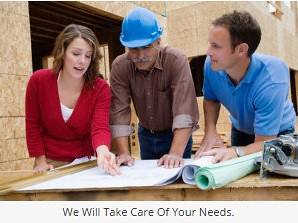In an advertisement image set at a construction site, three individuals are seen closely examining architectural plans spread out on a table. The background showcases the skeleton of a house under construction, with its unfinished wooden frames exposed. On the left stands a young white woman in her 20s, wearing a red long-sleeve shirt, her shoulder-length brown hair framing her face as she points decisively at the blueprints. Her mouth is slightly open, indicating she is speaking. In the middle, an older man, likely the builder, dons a blue hard hat. He sports a gray mustache and is dressed in a button-down shirt with the sleeves rolled up and jeans. His eyes follow the woman's pointing finger, fully engaged in the discussion. To the right, another man with short brown hair leans over the table, wearing a light blue polo shirt. He seems to be listening attentively to the woman. The table is cluttered with rolled-up blue and green papers, adding to the scene's authenticity. At the bottom of the image, a caption reads, "We will take care of your needs," underscoring the collaborative and attentive nature of their work.